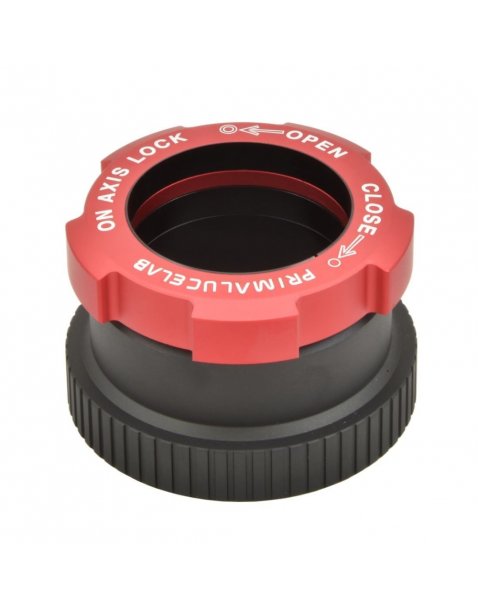The image depicts a black and red cylindrical object, likely a specialized cap, lock, or lens component, set against a plain white background. The black base features perforations around its circumference, while the top part is a red metal ring adorned with white lettering. The text on the red ring reads "ON AXIS LOCK," followed by an arrow pointing left with the word "OPEN," and another arrow pointing right with the word "CLOSE." There is also the text "PRIMALUCELAB" on the red ring, though the exact wording is challenging to discern. The object's purpose is ambiguous, but it appears to be some sort of locking mechanism or cap, given its structured design and labeling.